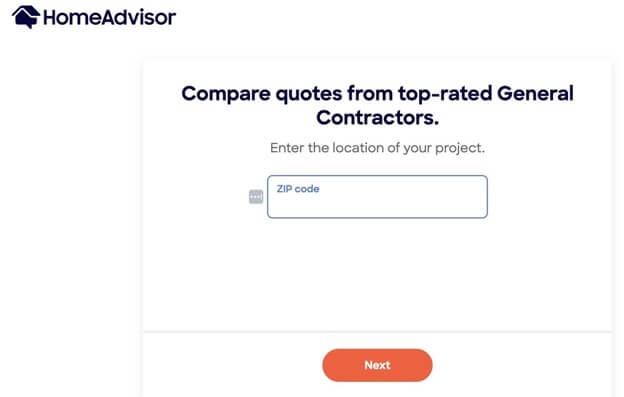The image is a web page for HomeAdvisor with a clean, white background. In the top right corner, a blue icon depicts a house with a roof, symbolizing the HomeAdvisor brand. Beside the icon, the word "HomeAdvisor" is written, with a capital 'H' and 'A' and the rest in lowercase letters.

Centrally positioned on the page, a prominent blue headline reads, "Compare Quotes from Top-Rated General Contractors." The words "Top-Rated" are separated by dashes. Below this headline, in smaller, gray text, it prompts users to "Enter the Location of Your Project."

A blue-outlined rectangle serves as an input field for the zip code. In the top left corner of this input field, the label "ZIP Code" appears, with 'ZIP' in capital letters and 'Code' in lowercase.

Further down the page, a thin gray line separates the input field from a large, eye-catching button. This button is shaped like a rounded rectangle, colored in orange, with the word "Next" in white, featuring a capital 'N' and the remaining letters in lowercase.